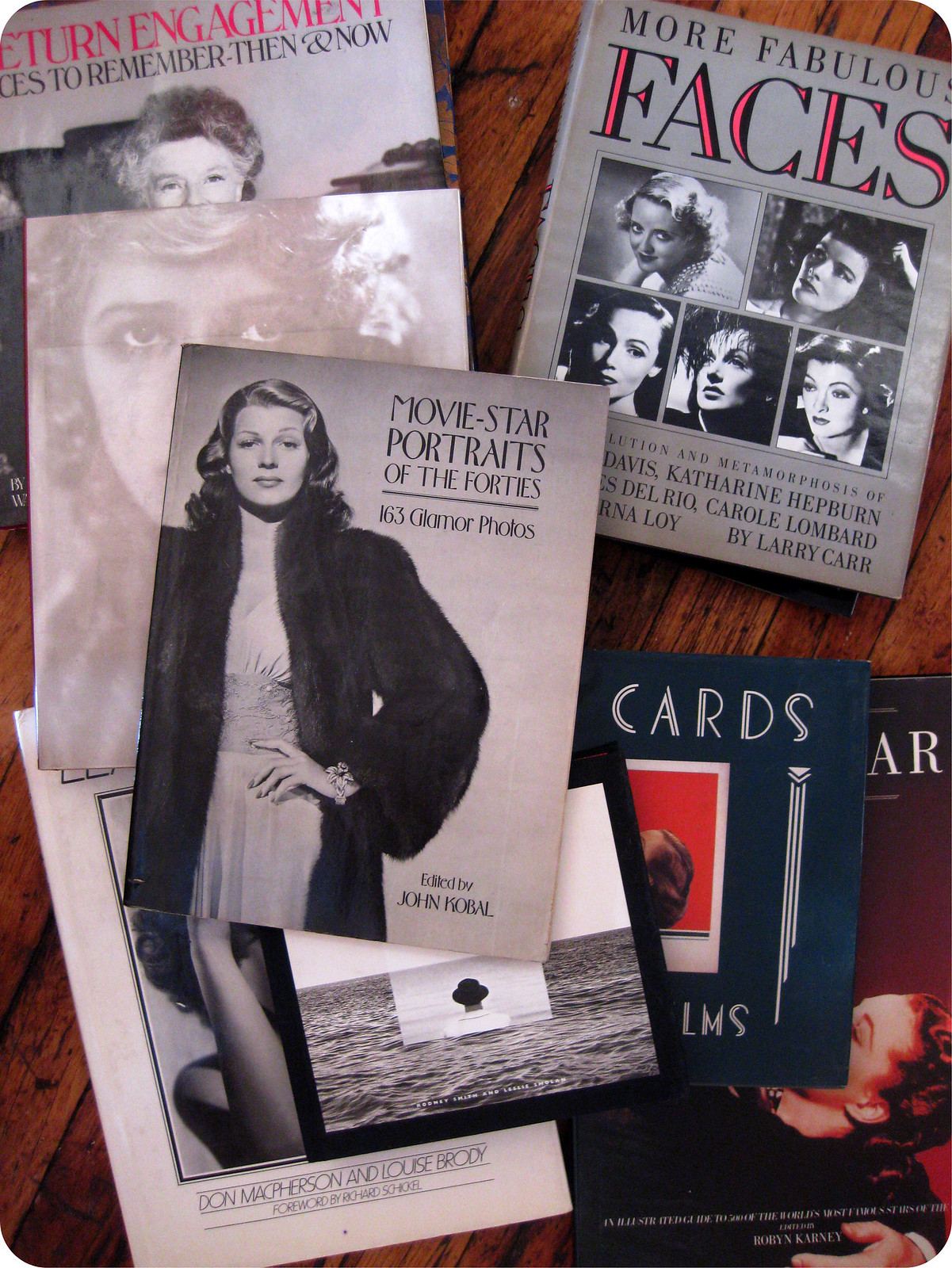The photograph displays a collection of six or seven books and magazines laid out on a dark wooden surface, perhaps a table or floor, giving a rich backdrop to the scene. The majority of the book and magazine covers feature black and white photographs of women, exuding a vintage Hollywood glamour theme. The most prominent book, positioned at the top of the pile, titled "Movie Star Portraits of the 40s," showcases an image of an elegant woman with glamourously styled dirty blonde hair. She is wearing a long fur coat over a light-colored gown, her left hand resting on her hip. The book also mentions it was edited by John Kobal, featuring '163 glamour photos.' Among the other covers, there's one called "More Fabulous Faces," set against a gray background and depicting five different actresses, with names like Katharine Hepburn and Carole Lombard. Sprinkled among these are a few color covers, notably situated towards the bottom right corner of the arrangement. Some book covers are partially obscured, mentioning only words like "cards," suggesting additional themed publications. This collection captures the essence of vintage Hollywood, celebrating its iconic leading ladies.